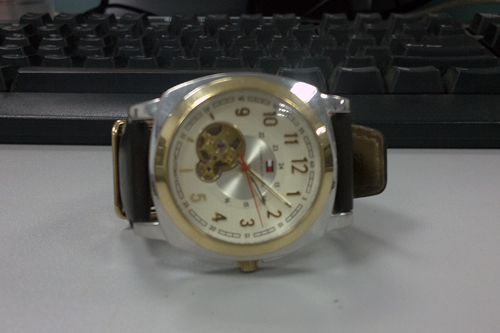This image features a close-up of an elegantly designed wristwatch with intricate details. The watch is mounted on a dark brown leather strap, accentuating its sophisticated silver case. The bezel, a blend of silver and gold, frames a pristine white dial. Gold numerals from 1 through 12 demarcate the hours, providing a striking contrast against the dial. At the center of the watch, a silver circle hosts a red and white emblem, adding a unique touch. Encircling this emblem are numbers ranging from 0 to 24. The watch hands are finely crafted in gold for the hour and minute, complemented by a slender red second hand. On the left side of the watch face, several small, indented gold discs are noticeable, though their purpose is unclear. The watch itself is placed on a gray table or counter, with a black keyboard visible in the background, adding a modern yet understated context to the scene.